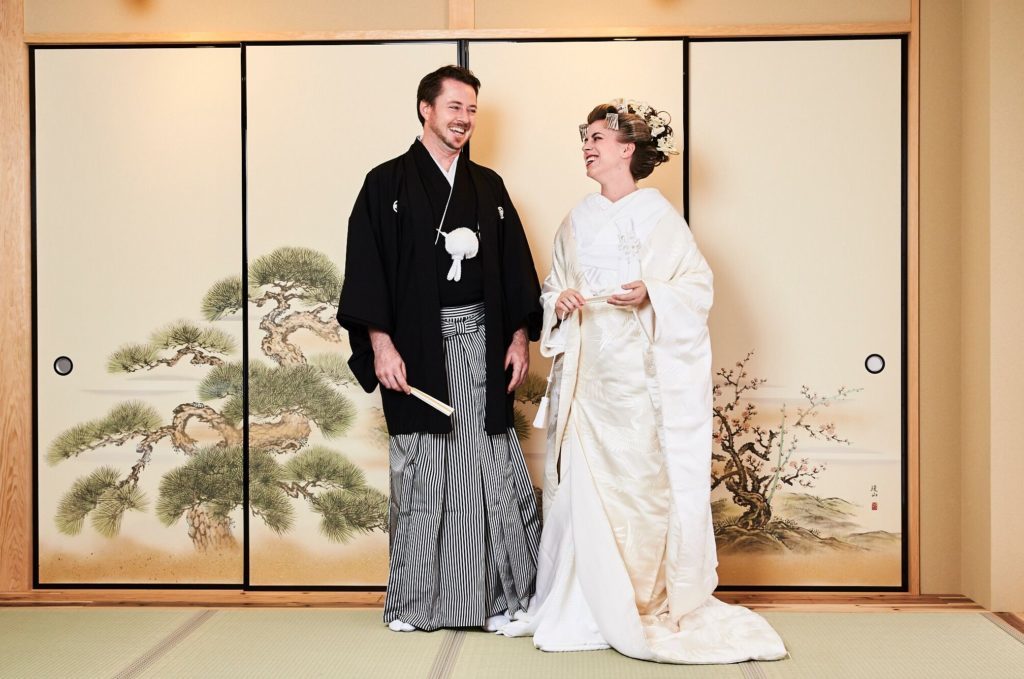In the center of the image, a Caucasian man and woman, possibly in their late 20s or early 30s, are smiling and laughing as they face each other. The man, standing on the left, wears a black men's style kimono with a white ball design hanging from his neck and the bottom half featuring black and white stripes. He also has brown hair, a chin strap beard, and a mustache. In his right hand, he holds a hand fan. The woman, standing to his right, is dressed in a flowy, all-white kimono. She has dark brown hair styled in a traditional Japanese manner, adorned with flowers, resembling a floral headdress. Her makeup includes lipstick, complementing her slightly paler complexion.

They stand in front of a Japanese-style wall with sliding doors, framed by black edges. The doors exhibit traditional Japanese paintings, including green-leaved bonsai trees on one side and ones with smaller, thinner leaves on the other. The pale yellow sky forms the backdrop of the paintings. The doors have handles encircled by black rings located on the far left and right sides, adding to the traditional aesthetic. This scenic setting and their attire suggest the possibility of this being a wedding photo or a portrayal of traditional Japanese costumes.